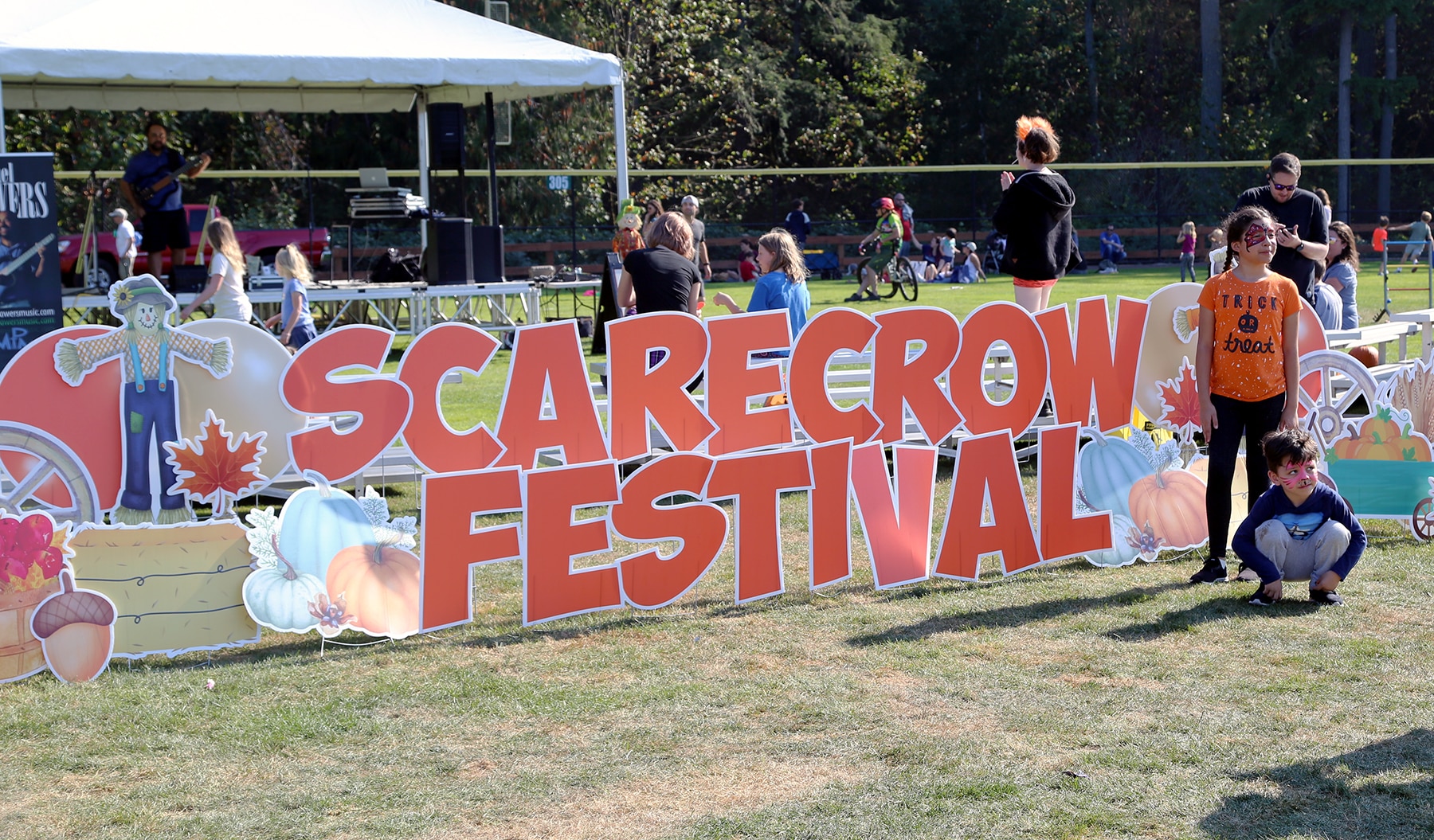The photograph captures a lively scene at the "Scarecrow Festival." Dominating the bottom two-thirds of the image is a vast, grassy area, with some sections appearing lush and green while others are dry and brown. The upper third is filled with dense, dark green trees, mainly clustered on the right side. In the central foreground, a large, eye-catching banner with red, uppercase letters reads "Scarecrow Festival." To its left, cardboard cutouts of a scarecrow, pumpkins, acorns, and perhaps an onion add to the festive atmosphere. 

To the left of the banner, a white tent shelters a stage where a performer, barely visible, appears to be playing a guitar amidst sound equipment. A few audience members are visible near the stage, with some approaching it while others engage in different activities, oriented away from the stage. Notably, two young children are posing for photos near the banner; one girl in an orange "Trick or Treat" t-shirt and black pants stands, while a boy in a dark blue t-shirt and light blue jeans sits beside her. The overall scene is animated with festival-goers enjoying the event, framed by the natural and festive decorations.